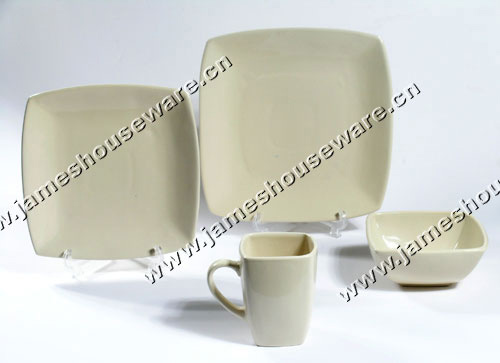The image features a collection of white dishware items set against a background that transitions from a light bluish-gray at the top to white at the bottom. On the left side of the image stands a square-shaped plate with slightly pointed corners, displayed on an acrylic stand. Adjacent to this, slightly higher and to the right, is a larger square plate of similar design. Towards the right of the image, placed on the surface, is a square-shaped bowl with rounded-off corners. In the center foreground, there is a square-shaped coffee mug with a handle on the left, appearing empty. The entire scene casts clear shadows on the surface below. Superimposed diagonally across the image, in white letters, is the URL "www.jameshouseware.cn," repeated three times from the top left to the bottom right.